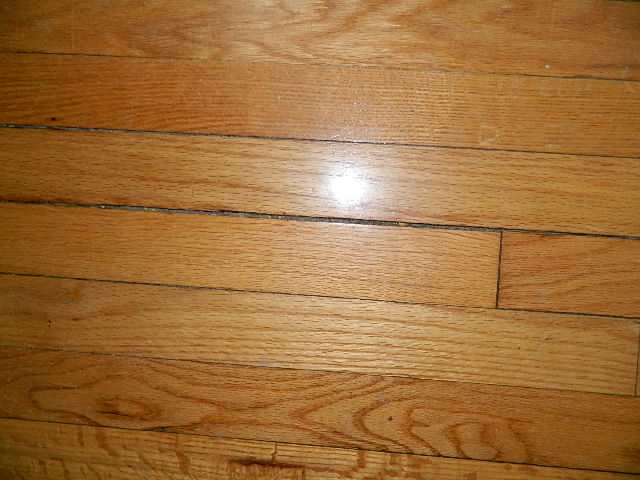The image depicts a floor composed of light brown wood panels, meticulously arranged in a square pattern. The natural grain of the wood is clearly visible, showcasing intricate lines and oval shapes characteristic of genuine timber. A light source casts a gentle reflection on the surface, accentuating the texture and enhancing the visual depth of the wood. The overall scene highlights the beauty and craftsmanship of the wooden flooring.